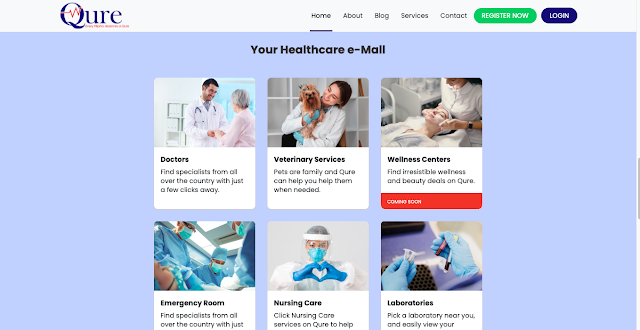Below is a cleaned-up and detailed caption for the given image:

---

This image is a screenshot of a healthcare-oriented website named "Qure," spelled Q-U-R-E, featuring a red, lifeline-style logo integrated into the Q. The upper-left section prominently displays the branding. The navigation menu includes links to Home, About, Blog, Services, and Contact, with a green "Register Now" button and a blue "Log In" button to the right.

The central area has a blue background with black text prompting the user, "Your Healthcare Email." Below this prompt, the webpage features six distinct images with corresponding service categories:

1. **Doctors**: An image of a man in a white lab coat engaging in a discussion with a woman wearing a pink sweater. The caption reads, "Find specialists from all over the country with just a few clicks away."
2. **Veterinarian Services**: A woman in a lab coat gently holding a dog. The caption highlights, "Pets are family. Cure can help you help them when needed."
3. **Wellness Centers**: Although the image details are not provided, the caption teases upcoming offers: "Find irresistible wellness and beauty deals on Cure coming soon."
4. **Emergency Room**: The image detail is missing, and the caption appears to be cut off after, "Find specialists for all over the country with just..."
5. **Nursing Care**: The specific image isn't detailed, but the partial caption states, "Click Nursing Care Services on Cure to help."
6. **Laboratories**: The truncated caption reads, "Pick a laboratory near you and easily view your..."

Overall, the website supports comprehensive healthcare needs with an easy-to-navigate interface.